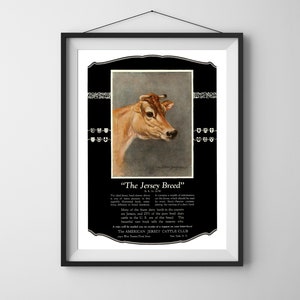Displayed prominently on a blank white wall, this detailed and intricately framed artwork features the image of a young light brown Jersey bull. The bull, shown from the shoulders forward, has striking black eyes, a black snout, and small forward-pointing horns. The photograph is encased in a sophisticated, multi-layered black frame that includes a delicate inner plaque. This plaque highlights the breed name "Jersey" in white text against a black background. Beneath this, there is additional text that remains unreadable due to its fine print. The bull's image is set against a backdrop composed of shades of gray and white, meticulously detailed to emphasize the breed's distinct characteristics. The frame is secured to the wall by a visible nail and wire, adding a touch of rustic charm to the otherwise elegant presentation.